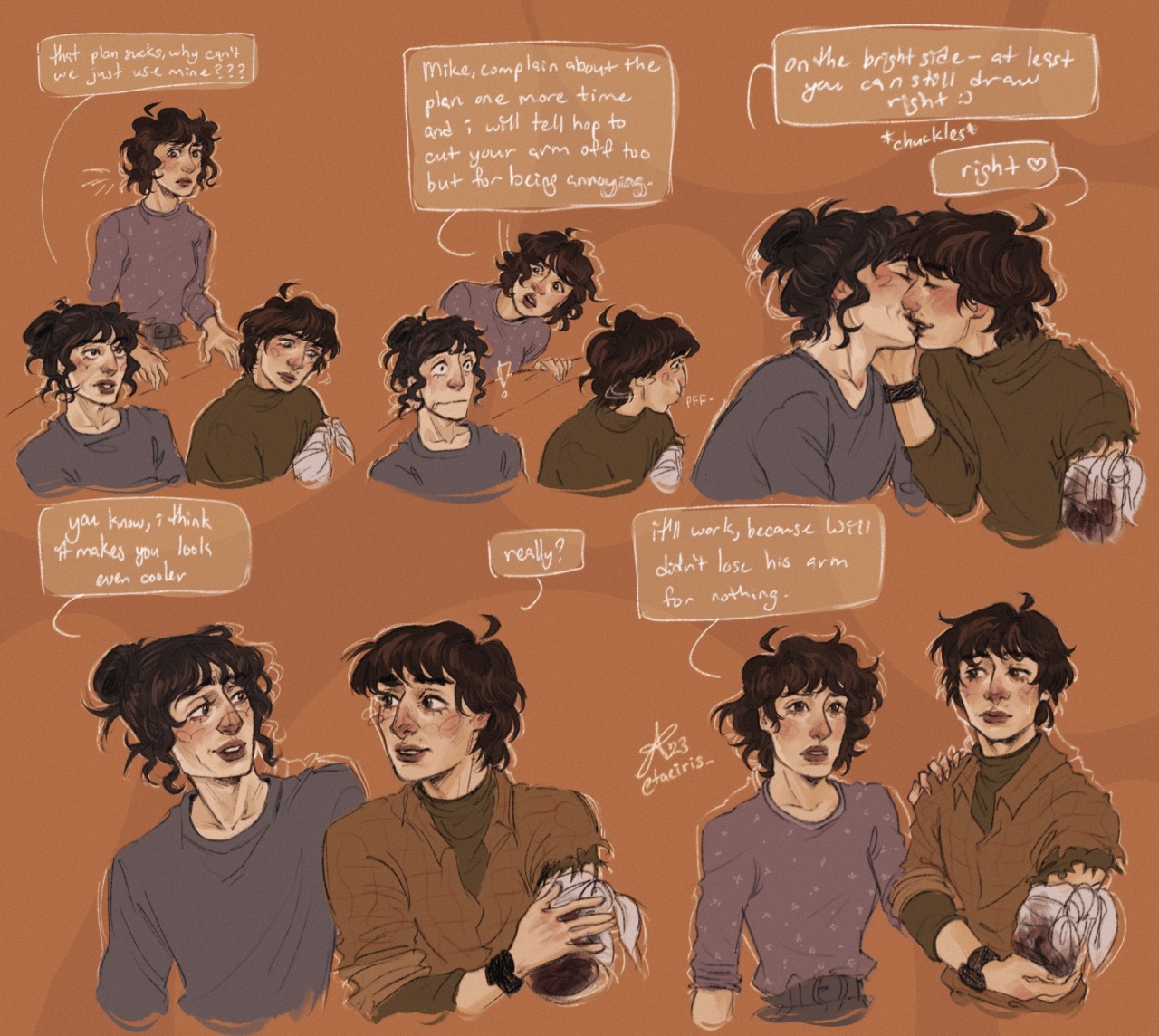The image features a series of cartoon panels displayed from top to bottom, progressing left to right. The background is a blend of brown and tan hues. There are two primary characters—a man and a woman—alongside a secondary character who occasionally appears to make comments.

In the first panel, positioned at the top left, the man and woman are depicted. The man is wearing a brown shirt, and the woman is dressed in a gray shirt. The woman, situated slightly in the background, is suggesting her plan by saying, "That plan sucks. Why can't we just use mine?" The man appears sad in response to her comment.

In the next panel, the man responds sternly, “Complain about the plan one more time, and I'll tell Hap to cut your arm off for being so annoying.” The woman is visibly shocked by this statement. Meanwhile, she tries to lighten the mood by saying, "On the bright side, at least you can still draw, right?" and chuckles. The man replies with a 'Right,' and they share a passionate kiss.

In the concluding panel, the woman comments, "You know, I think it makes you look even cooler with a bloody arm cut off." The man, somewhat taken aback, responds, "Really?" She affirms, "Yes, because, well, we didn’t lose his arm for nothing." The man appears thoughtful, considering the strangeness of their situation.